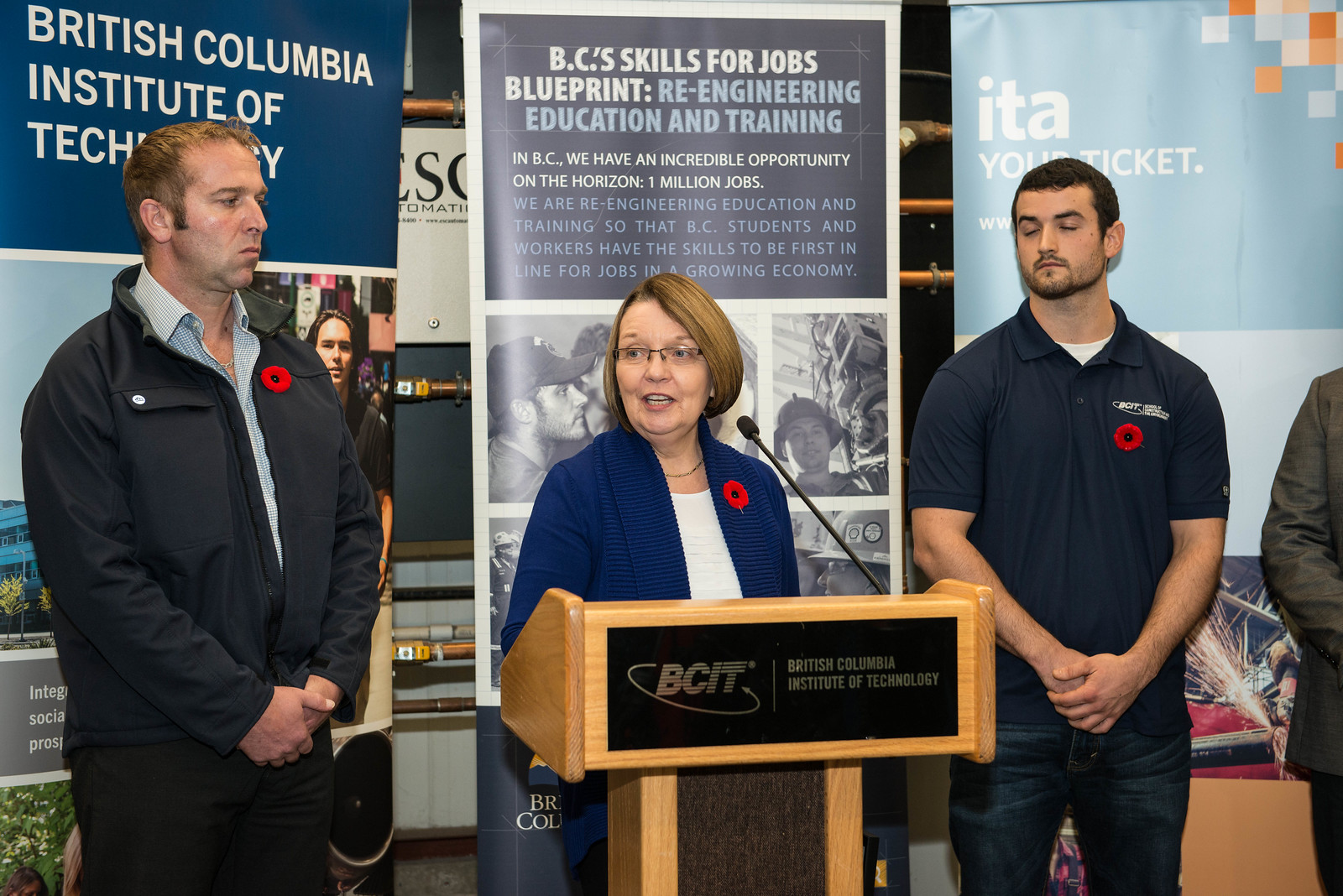This photograph, taken indoors, features a woman standing at a wooden podium with the logo of the British Columbia Institute of Technology (BCIT) prominently displayed. The woman, who appears to be middle-aged with short brown hair and glasses, is wearing a blue jacket over a white undershirt, accented by a red flower pinned to her jacket. She is turned slightly to her left as she speaks into the microphone positioned in front of her. To her left stands a man dressed in dark brown pants, a dark jacket, and a blue and white undershirt, similarly adorned with a red flower. To her right, another man stands directly next to her, dressed in a blue shirt and blue pants with a flower pinned to his attire as well. Partially visible behind her on the right is a third man wearing a suit. 

The background is filled with banners displaying various messages, including "British Columbia Institute of Technology," "ITA," "Your Ticket," "BC Skills for Jobs Blueprint," and phrases like "Reengineering Education and Training" and "We have an incredible opportunity on the horizon – 1 million jobs. We are re-engineering education and training so that BC students and workers have the skills to be first in line for jobs in a growing economy."